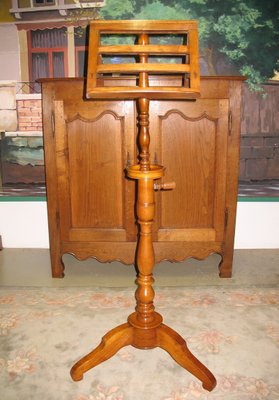This photograph captures a detailed scene set on what appears to be a balcony or a patio area outside a building. In the foreground stands a walnut-colored wooden music stand, complete with an adjustable telescoping base and three feet reminiscent of a coat rack, placed on a floral-patterned rug. Behind the music stand, there is a two-door hutch-style cabinet, seemingly from the 1950s or early 1960s, with a flat surface on top. The music stand obscures the center of this medium brown cabinet, making the details of its doors partially hidden. Beyond these pieces of furniture, the scene expands into an outdoor setting, revealing a light tan or light peach stone building in the distance and the foliage of a tree. A wooden fence divides this outdoor space, where additional elements like a brick wall, possibly some windows with an awning, and ambiguous objects that might be trash cans are faintly visible, adding layers of complexity to the setting.